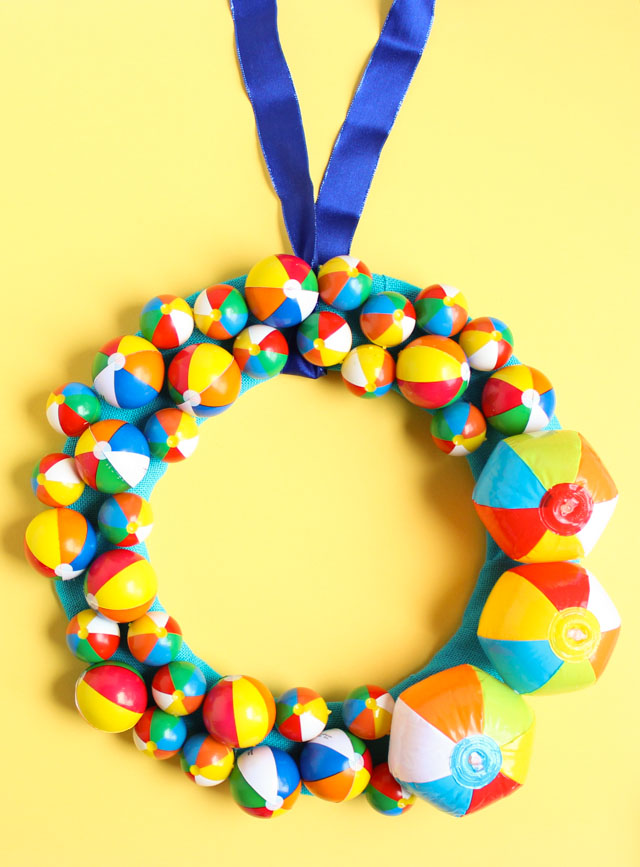The image features a pastel yellow background with a prominent circular wreath at the center, resembling a lifesaver in size and shape. This wreath, primarily light blue, is adorned with numerous beach balls of various sizes, primarily small but with three larger ones creating a focal point on the middle and bottom right. The beach balls are vibrantly colored in a mix of white, blue, orange, yellow, red, and green, each with a central white circle. Two blue ribbons, starting from the top of the image, descend in a V-shape and connect to the wreath, adding a sleek visual element to the ensemble.